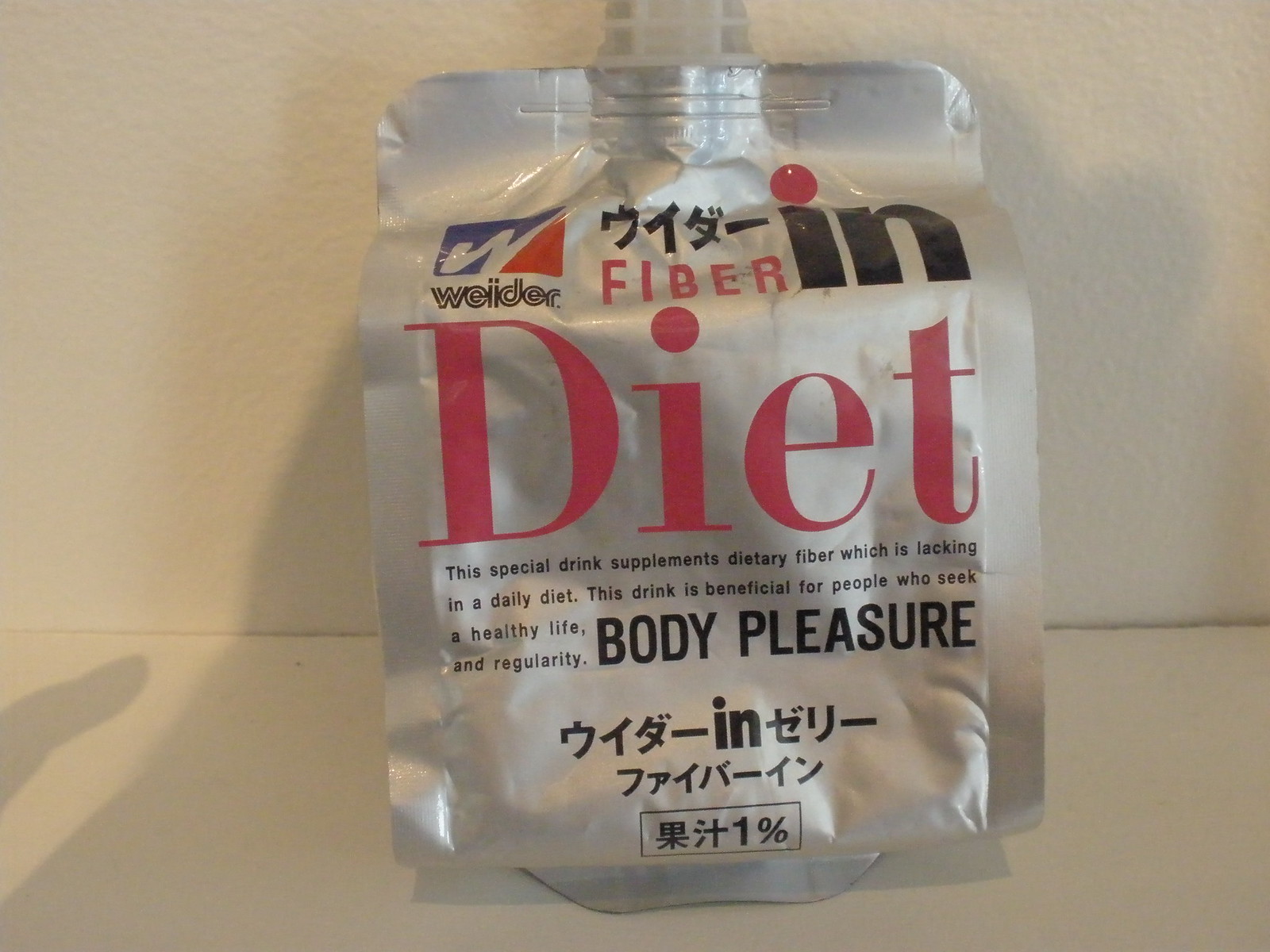The image features a silver-colored package set against a white backdrop, both beneath and behind the product. The backdrop exhibits a slight stippling effect, suggesting it might be a painted wall. A faint shadow is present, likely cast by the photographer. The package includes a cut-off white plastic spout at the top, indicating it could be used for drinking. The front of the package prominently displays the brand name "Weider" and the product name "Fiberin." The word "Diet" is highlighted in large pink letters. Below, the text reads: "This special drink supplements dietary fiber, which is lacking in daily diet. The drink is beneficial for people who seek a healthy life, body pleasure, and regularity." Additionally, there are several characters in Japanese on the package.